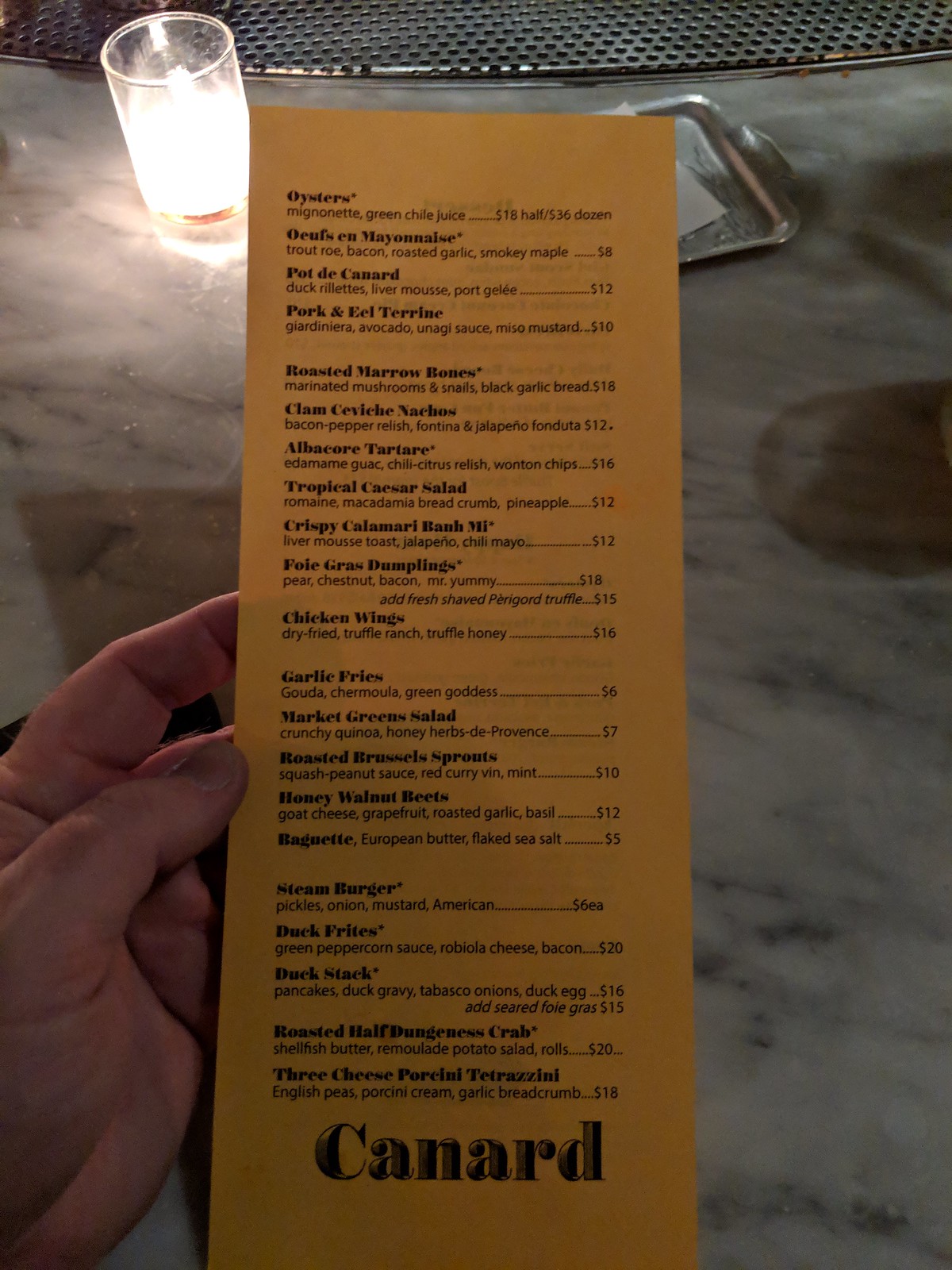In this slightly dark, color photograph taken outdoors, a thin, rectangular, orange menu is prominently featured. The photo, captured in portrait mode, shows the menu being held on the left side by a hand with light-colored skin. The background reveals a white table with a distinctive black marbling pattern. A small candle, housed in a glass resembling a drinking glass, is lit, adding a warm glow to the scene. Partially visible behind the menu is the edge of a small green tray.

The menu itself bears the restaurant name "Canard" in large black type at the bottom. It features a list of appetizers, each item titled in bold type with descriptions and prices detailed underneath in regular type. At the bottom of the menu, several meal choices are listed, including burgers, fries, duck, crab, and tetrazzini.